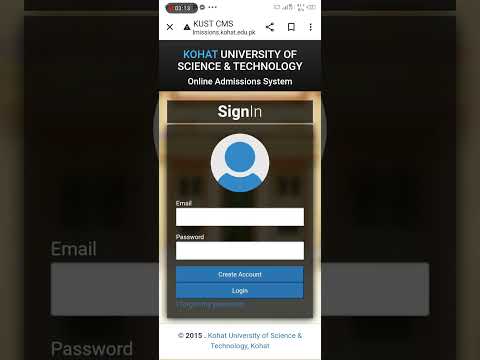On a black background, a simulated mobile phone screen is displayed, capturing the essence of a website's interface. The top-left corner features the number "313" in white lettering. Adjacent to this, a circular gray icon and three gray dots are positioned, followed by a gray "X" and a gray triangle.

Further to the right, the text "K-U-S-T C-M-S" appears in gray, capital letters. The typical Android share icon—a right-pointing arrow with dots at the edges—is located next to a bookmark icon and a set of three vertical dots indicating a dropdown menu. The interface is bordered by a black rectangle.

Inside this rectangle, "KOHAT" is prominently displayed in blue, capital letters. Directly below, "University of Science and Technology" is written in all caps with white font, followed by "online admission system" in regular, lowercase white font.

The screen then transitions to a sign-in page. The word "Sign" is written in bold, capital letters, seamlessly continuing with "in" in unbolded letters without any spacing. Below this, a beige divider line is visible. A circular icon featuring a silhouette of a person is displayed prominently above the input fields for email and password.

At the bottom of the screen, two long, skinny blue rectangles stand out, filled entirely with blue. The left rectangle reads "create account" in white lettering, while the right rectangle reads "log in" in similar white lettering, guiding users towards their respective actions.